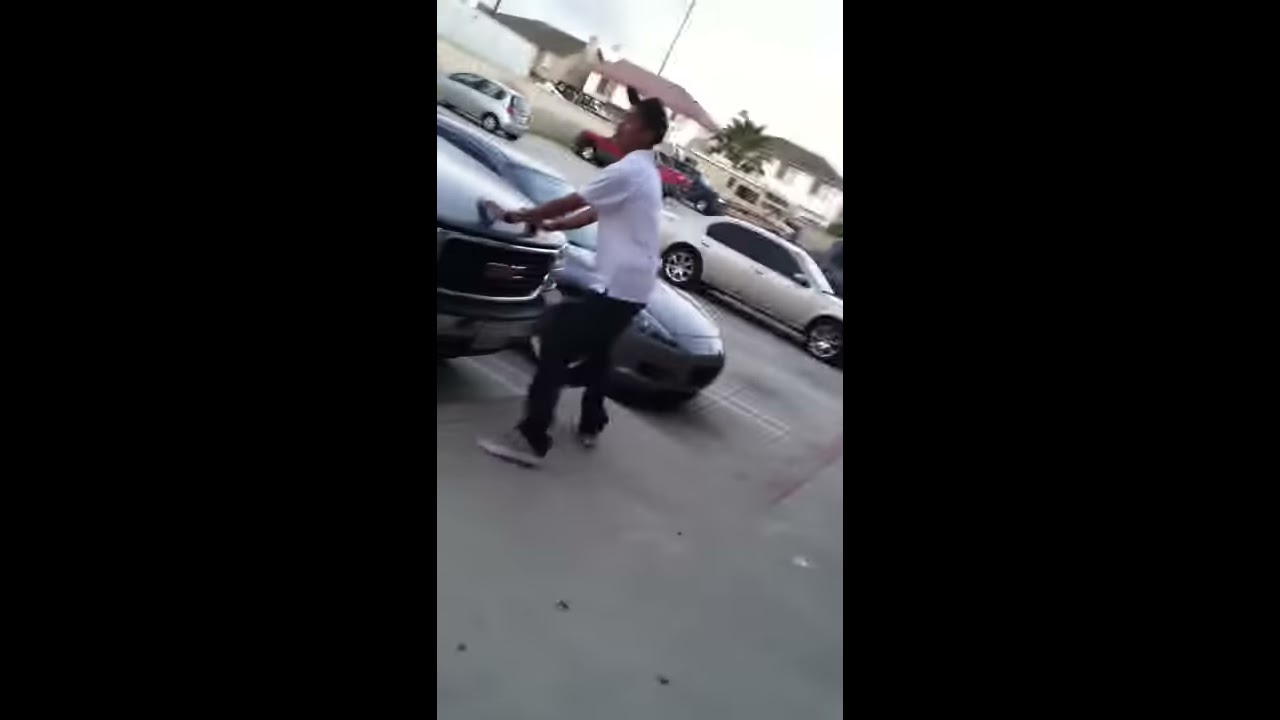In the image, we observe a man standing outdoors in a small parking lot, surrounded by a variety of vehicles and residential features. The man, who has darker skin, is dressed in a white shirt, black pants, gray shoes, and a flat cap. He appears to be pressing his hands against the front of a GMC truck, which is partially visible. To the right of this truck is a sporty black car, likely a Corvette, followed by a gray car in a parking space. The background reveals an RV with a yellow hue and decorative decals, a number of cars with tinted windows, and distant houses with a prominent palm tree. The overcast sky above is mostly white with some clouds, giving a bright but diffused lighting to the scene. The man is standing on gray asphalt, and there is a concrete wall visible along with an entrance. The image seems to be a still frame from a video, framed with left and right thirds filled with black bars, and has a tilted perspective making the elements appear as if they might slide to the bottom right.